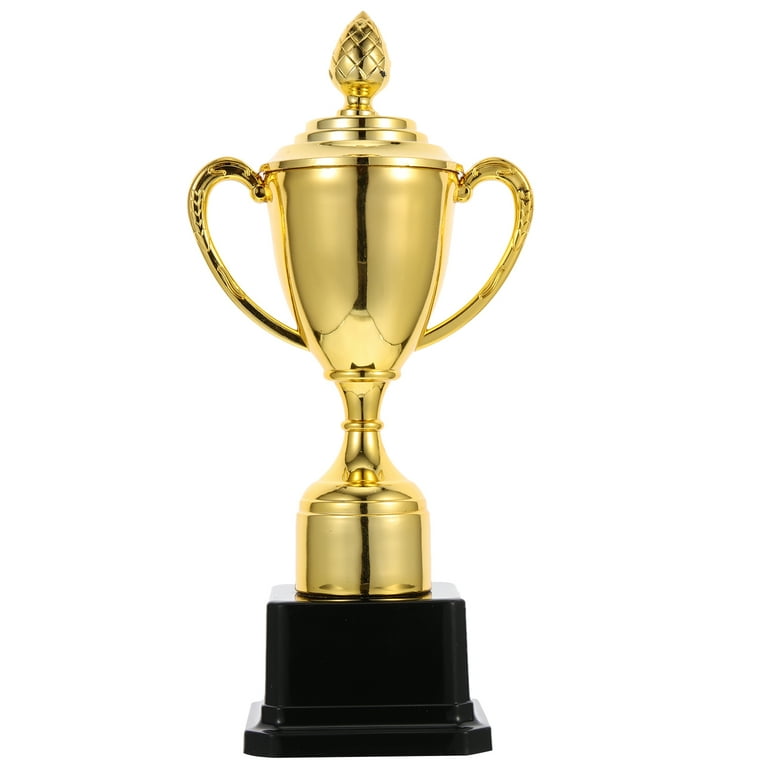The image displays a striking, large trophy set against a solid white background, ensuring all attention is on the trophy itself. This traditional-looking trophy, standing about 5 inches tall on its black, slightly layered base, is made of a highly reflective golden metal. The trophy boasts a classic goblet shape with two substantial golden handles extending from its sides. At the top, an ornament resembling an acorn or pine cone adds intricate detail. The body features a dark, squiggly line running from the ornamentation down to the base, which is black and seems to be crafted from a substantial plastic material. This elegant trophy, lacking any inscriptions or writing, epitomizes a classic award design with its bright, radiant gold finish and traditional form.